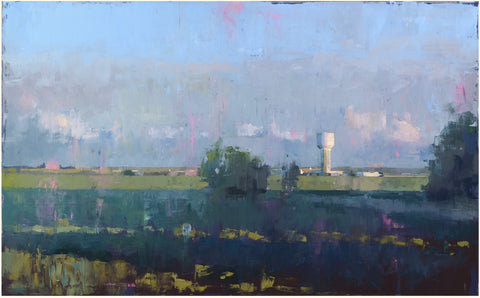This image conveys a detailed painting of a serene rural landscape, possibly created using acrylic or oil paints. In the foreground, a deep blue river or stream runs horizontally across the canvas, bordered by patches of light green grass in the bottom left corner. Along the far edge of the river, two large, bushy green trees stand prominently, framing the idyllic scene. Extending into the background, a lush, flat field of green grass or possibly wheat suggests the setting on a farm. A white silo and a large red-roofed barn sit near the right-center of the painting, accompanied by a white farmhouse with a black roof. The sky above the landscape is a calming light blue, adorned with soft white clouds, adding to the tranquil and pastoral atmosphere depicted in this detailed piece of artwork.